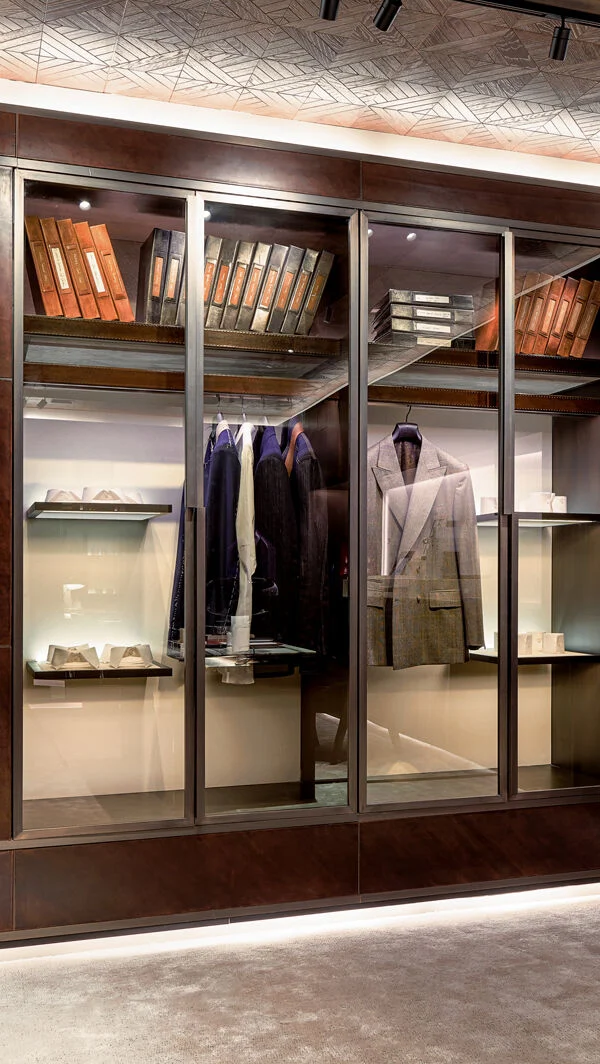This image captures a detailed view of a luxurious, well-organized men's closet, likely belonging to a professional or someone of high prominence. The closet features a rich, mahogany finish with top and bottom panes, and central floor-to-ceiling glass doors framed in dark silver metal, providing an elegant display of the contents. The plush taupe carpet adds a touch of warmth to the room. On the top shelf of the closet, several leather-bound binders, in shades of brown and black, offer a hint of the owner's importance. Below this shelf, there are two distinct sections: 

On the left side, we see four jackets—three in navy blue and one white shirt—all hanging neatly and viewed from the left shoulder. To the right, a clothing rack prominently displays a gray suit jacket, facing directly toward the viewer. The shelves to the left and right of the glass display cases hold white objects, possibly jewelry displays for watches and rings. The entire setup is impeccably organized, with the glass doors allowing for a clear and inviting view of the well-maintained wardrobe within this sophisticated, carpeted space.